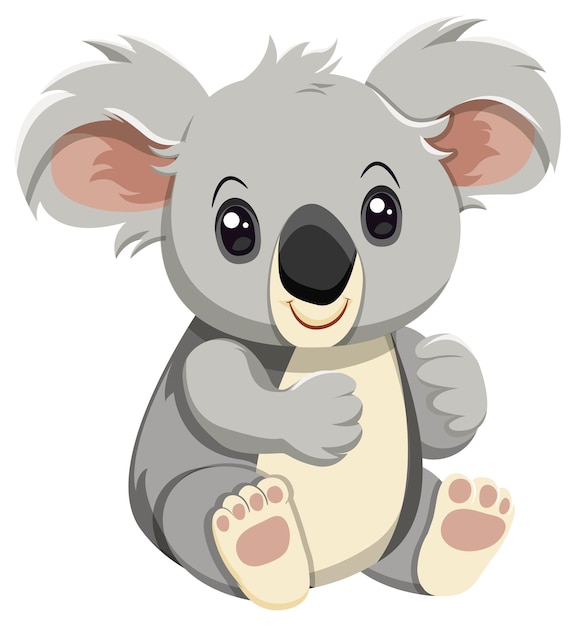A detailed cartoon illustration features an adorable koala bear sitting with its body facing towards the 5 o'clock position and its head tilted to look directly at the viewer. The koala, rendered in light gray, has a smiling face with big, buggy black eyes that have a twinkle and a prominent black nose. The ears are a pinkish flesh tone color with tufts of hair protruding. The koala’s belly is off-white or cream-colored, matching the area around its mouth and the bottom of its feet. The feet also reveal pink paw pads and darker, almost sandy-colored claws. Its arms are stretched out in front, seemingly ready to hug someone. This delightful koala’s design is reminiscent of a cute stuffed animal, accented by details like its pinkish ear interiors and the distinct colorations of its feet, adding to its charming, comforting appearance. The background is entirely white, giving no visual distraction from the koala itself.